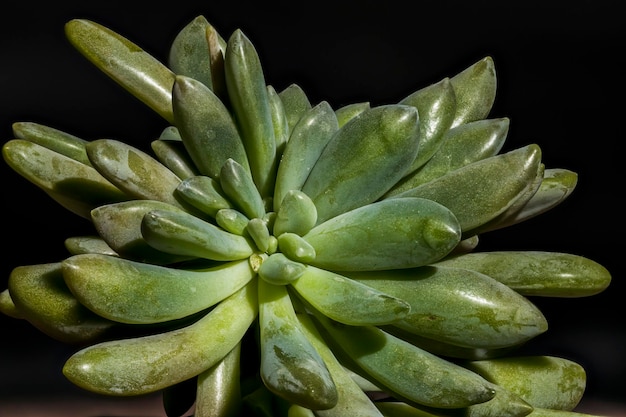This close-up image showcases a vibrant green cactus set against a stark black background. The cactus features long, banana-like leaves that are plump, shiny, and full, with a frosted, whitish appearance at the tips where the green color appears duller. The right leaves are noticeably thicker and more vibrant compared to the thinner and more spread-out ones on the left. The central part of the plant reveals smaller, not fully formed leaves that resemble green peapods bunched together, adding a unique textural element to the overall composition.